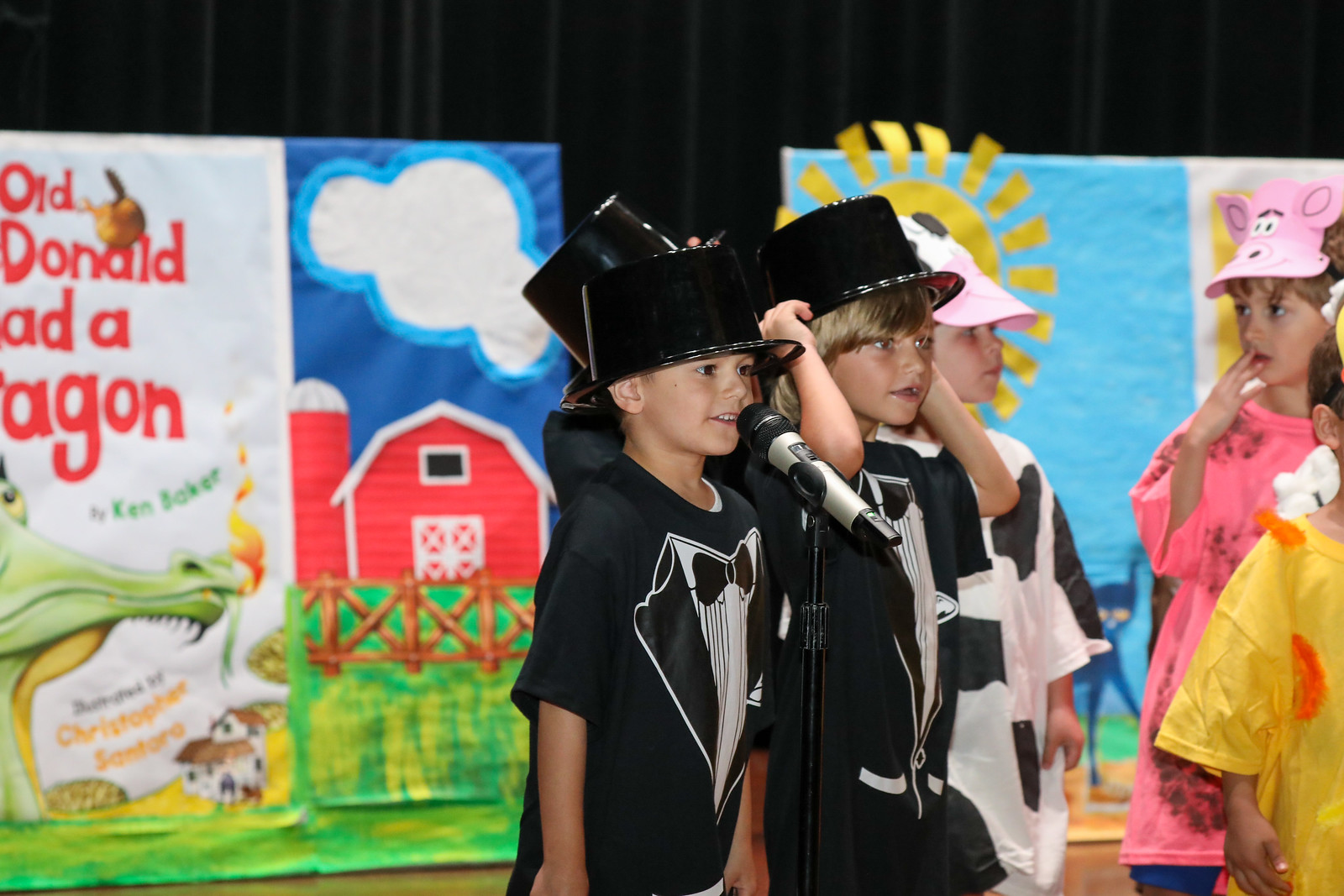This image captures a delightful scene from a children's play, "Old MacDonald Had a Dragon" by Christopher Santoro. On stage, against a backdrop of dark black curtains and hand-painted posters depicting a barn with a blue sky, a cloud, and a green dragon, six young children, around 7 or 8 years old, are performing. In the middle-right of the photograph, a little boy stands confidently at a microphone. He, along with two other boys, is dressed in a black tuxedo t-shirt complemented by plastic black top hats. Near them, scattered more to the right, are a few children dressed as farm animals. One girl with a pig mask and pink shirt holds her hand up to her face, while another child in a black and white costume wears a cap with a pink bill, seemingly portraying a cow. They stand slightly behind, adding a charming diversity to the scene. The lively homemade posters in the background, featuring a whimsical dragon and sunny barnyard elements, set a charming tone for the performance, hinting at the imaginative story being brought to life by these young actors.